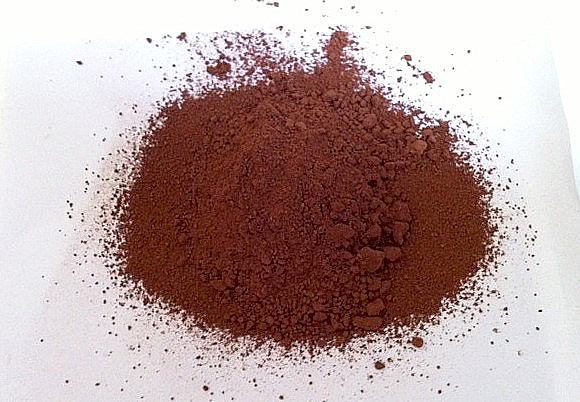The image depicts a cluster of chocolate-brown powder scattered across a white background, which appears to be a white cloth or sheet. The powder is largely concentrated at the center of the surface, with noticeable variations in particle size. Toward the top right and bottom right of the pile, the particles form larger clumps, while finer specks are dispersed around the perimeter of the pile. Additionally, the cloth shows slight folding on its right side.